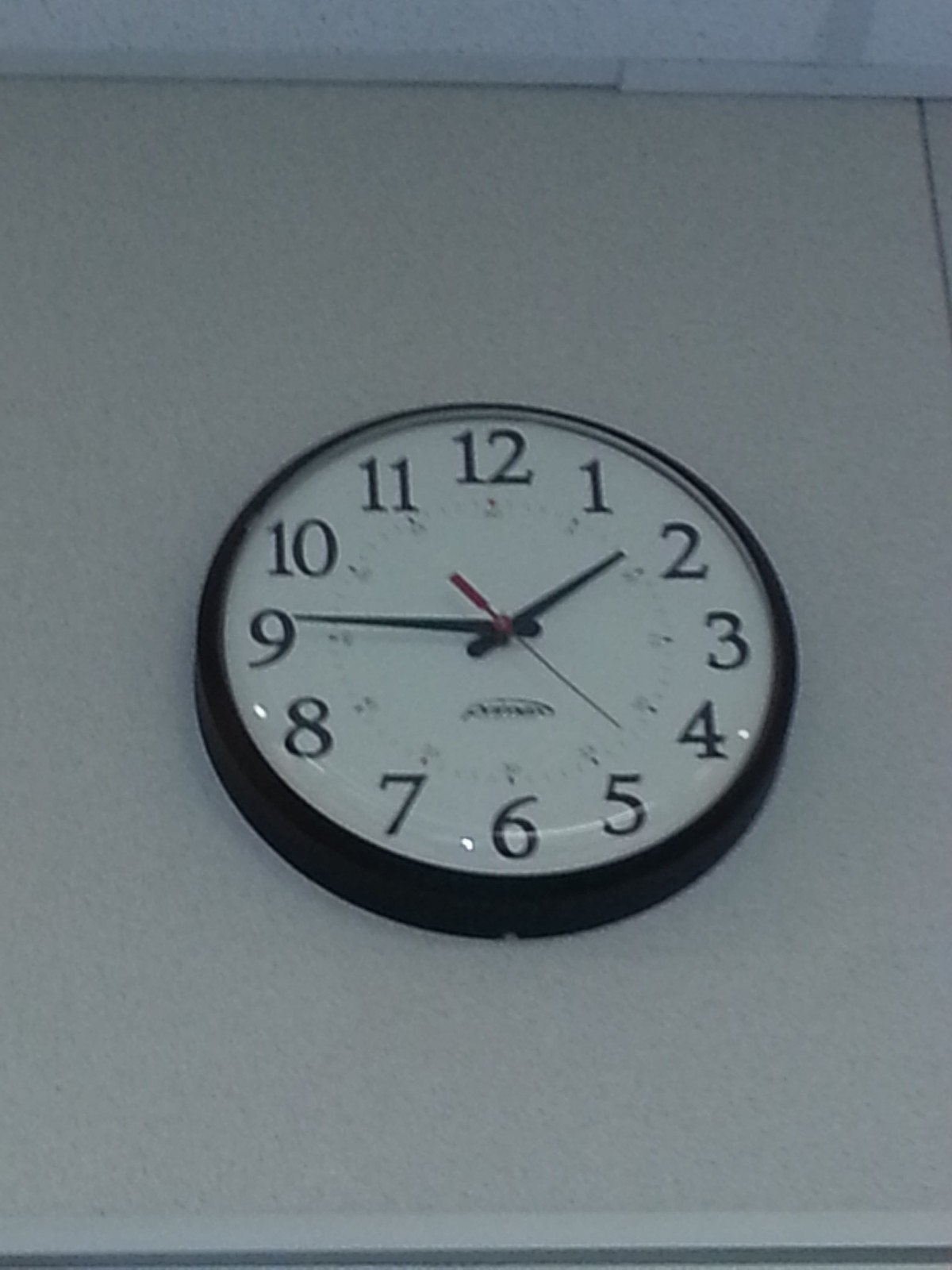This is an indoor color photograph, slightly blurry and grainy, taken looking up at a classic round analog wall clock. The clock hangs on a plain white wall, above a door frame, with part of a speckled plaster tile ceiling visible at the top of the image. The clock features a white face with large black numbers from 12 to 11, and black hour and minute hands. The second hand is red and positioned between the 4 and the 5, indicating the time is 1:45. The clock is set within a black outer bezel and protected by a glass cover which subtly reflects light in its lower portion. The overall lighting is dim, and the clock is seen at an angle, making the bottom part more prominent than the top. No text or additional markings are visible on the clock due to the slight blur and graininess of the image.